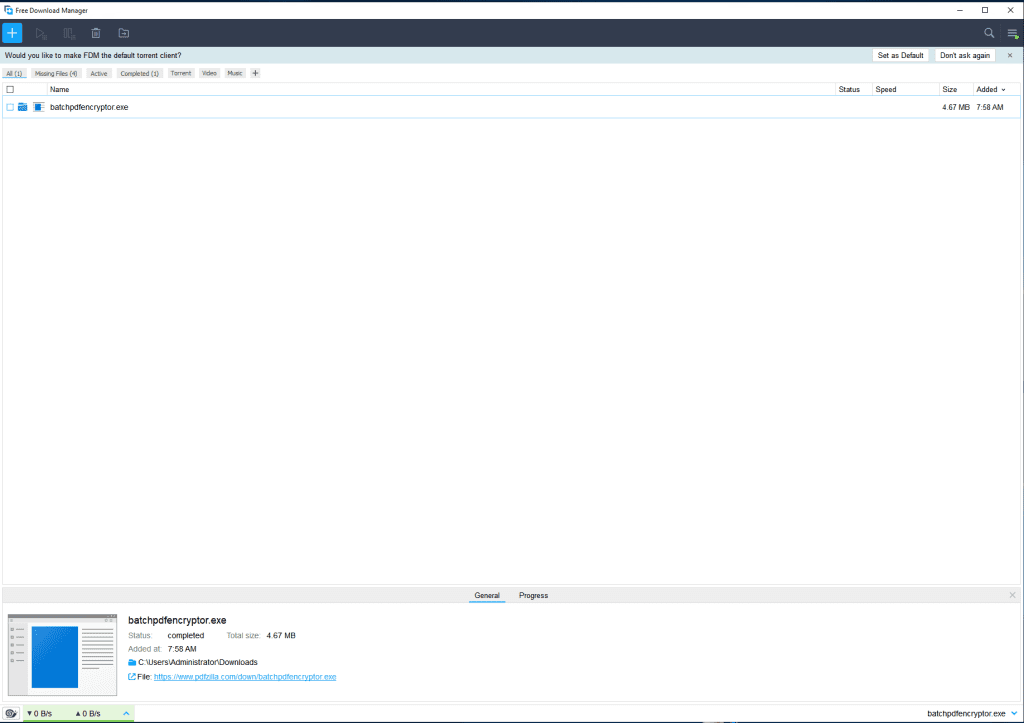The image prominently features a black banner at the top of the screen. In the upper left-hand corner of this banner, there is a blue square containing a plus sign and various icons aligned along the banner. Directly below this black banner, the text reads, "Would you like to take FDM, the default?" followed by an additional smaller, less readable text towards the center of the screen.

Directly beneath the confusing text, the word "Name" is displayed, followed by more text that is quite small and difficult to read. In the upper right-hand section of the screen, there are two options: "Set as default" and "Don't ask again." Directly below these options, there are labels for "States," "Speed," and "Size," accompanied by a tab labeled "Added" with a drop-down arrow beside it. Below this, the text reads "67 MBs" and the time is indicated as 7:58 AM.

While much of the central area of the screen is unoccupied, the bottom-left corner hosts a pop-up box with a blue square banner situated in its middle. Adjacent to this pop-up box, some additional text is displayed.